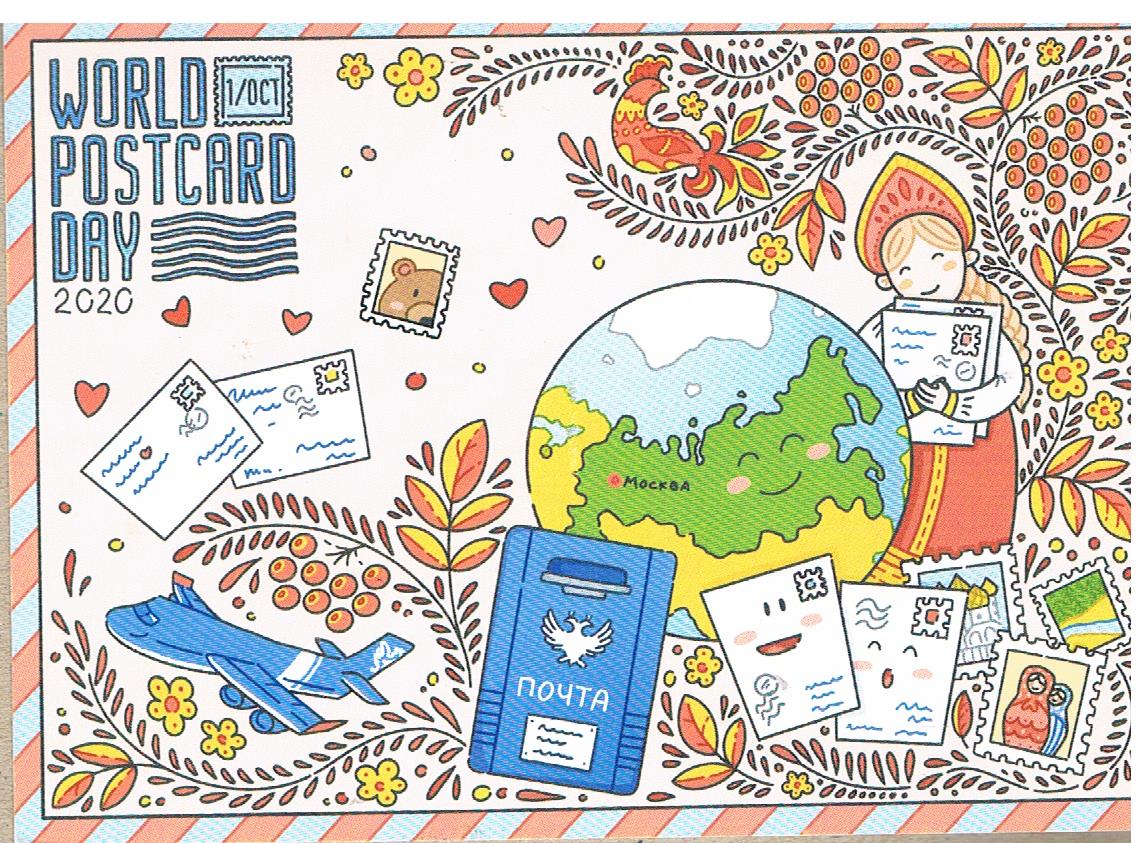This vibrant and colorful postcard, framed with light blue and orange stripes, creates the illusion of a postcard within a postcard. The main white background features a festive array of flying letters, postcards, and hearts, celebrating "World Postcard Day, 1 October 2020," prominently displayed in the upper left corner. A variety of playful illustrations such as a stamp with a bear, a blue airplane, a blue passport, and various letters are scattered throughout the scene.

At the heart of the postcard is a detailed circular image depicting a map, specifically highlighting Moscow, labeled as MOCK (in Cyrillic as M-O-C-K-B-A). Overlaid on this map is a cheerful, cartoonish girl dressed in a red traditional gown, seemingly embracing the world and clutching two postcards. Surrounding her is an exuberant collage of birds, flowers, leaves, and whimsical designs, enhancing the postcard’s lively and jovial atmosphere.

The lower left of the postcard showcases a blue airplane taking off, surrounded by small, round fruits or berries, and fern leaves. Additional decorative elements include postage stamps with diverse images—such as one depicting a brown bear—and a cascade of hearts mingling with the other illustrations, all contributing to the postcard's overall celebratory and busy theme.